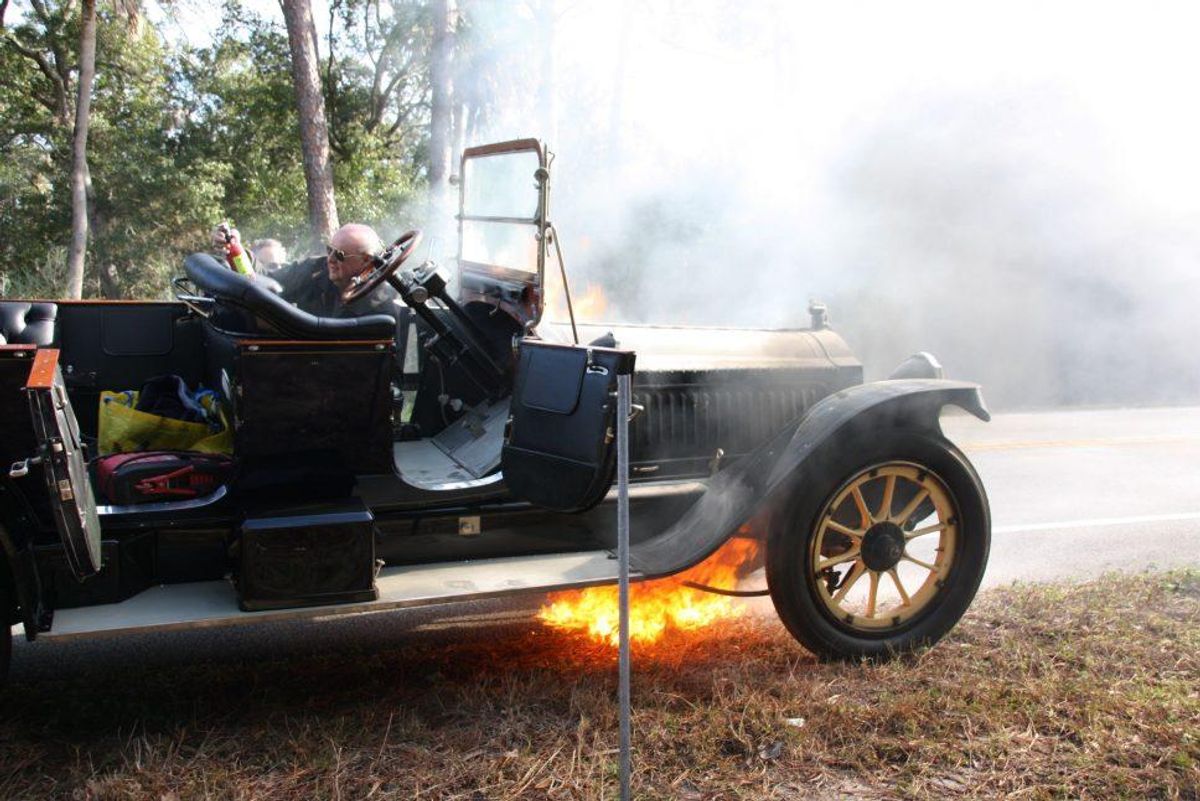The photograph captures a dramatic scene featuring a very old-fashioned, classic black car with a gold hood and matching gold-rimmed tires, reminiscent of a Ford T-Model. The car, devoid of a roof and with both its front and rear doors open, is stalled on the side of the road amid dead grass and various debris. The car is engulfed in flames underneath, with yellow and red flames visibly licking the bottom of the vehicle, and bellowing white smoke spiraling upward. 

A policeman, equipped with a fire extinguisher, is reaching into the car, presumably attempting to manage the blaze. Another man, who somewhat resembles Joe Biden and is wearing sunglasses, stands behind the vehicle on the road, smiling and seemingly unbothered by the fire. The setting includes a few trees in the background and a signpost missing its sign in front of the car. There's notable clutter on the back seat's floor and the front seats of the car, adding to the overall sense of disarray in the scene.